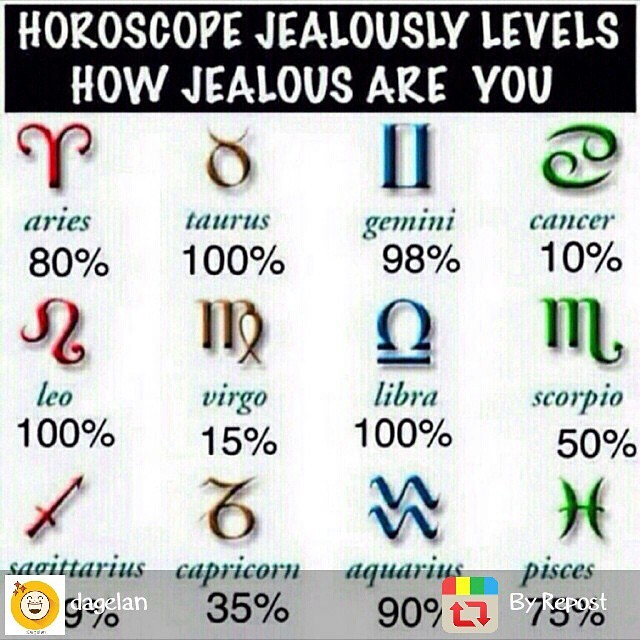The image showcases a "Horoscope Jealousy Levels" chart, presented within a black rectangular bar adorned with white, handwritten-style font. This chart quantifies the jealousy levels of each zodiac sign, organized in a 4x3 grid format. Each zodiac sign is represented by its symbol and name in four different colors: red for the first column, dark gold for the second column, blue for the third column, and green for the fourth column, with their jealousy percentages listed underneath in black font. The specific breakdown is as follows:

- **Top row**: Aries (80%), Taurus (100%), Gemini (98%), Cancer (10%)
- **Second row**: Leo (100%), Virgo (15%), Libra (100%), Scorpio (50%)
- **Bottom row**: Sagittarius (partially hidden by a sticker of the sun, showing "9%"), Capricorn (35%), Aquarius (90%), Pisces (75%)

Given the color-coded symbols, the Aries and Taurus entries stand out in their light green, the same as the remaining symbols in their respective columns. The background is a clean white, and at the bottom of the image are some branding elements: a logo for "Dage Land" on the lower left and "Buy Repost" on the lower right.